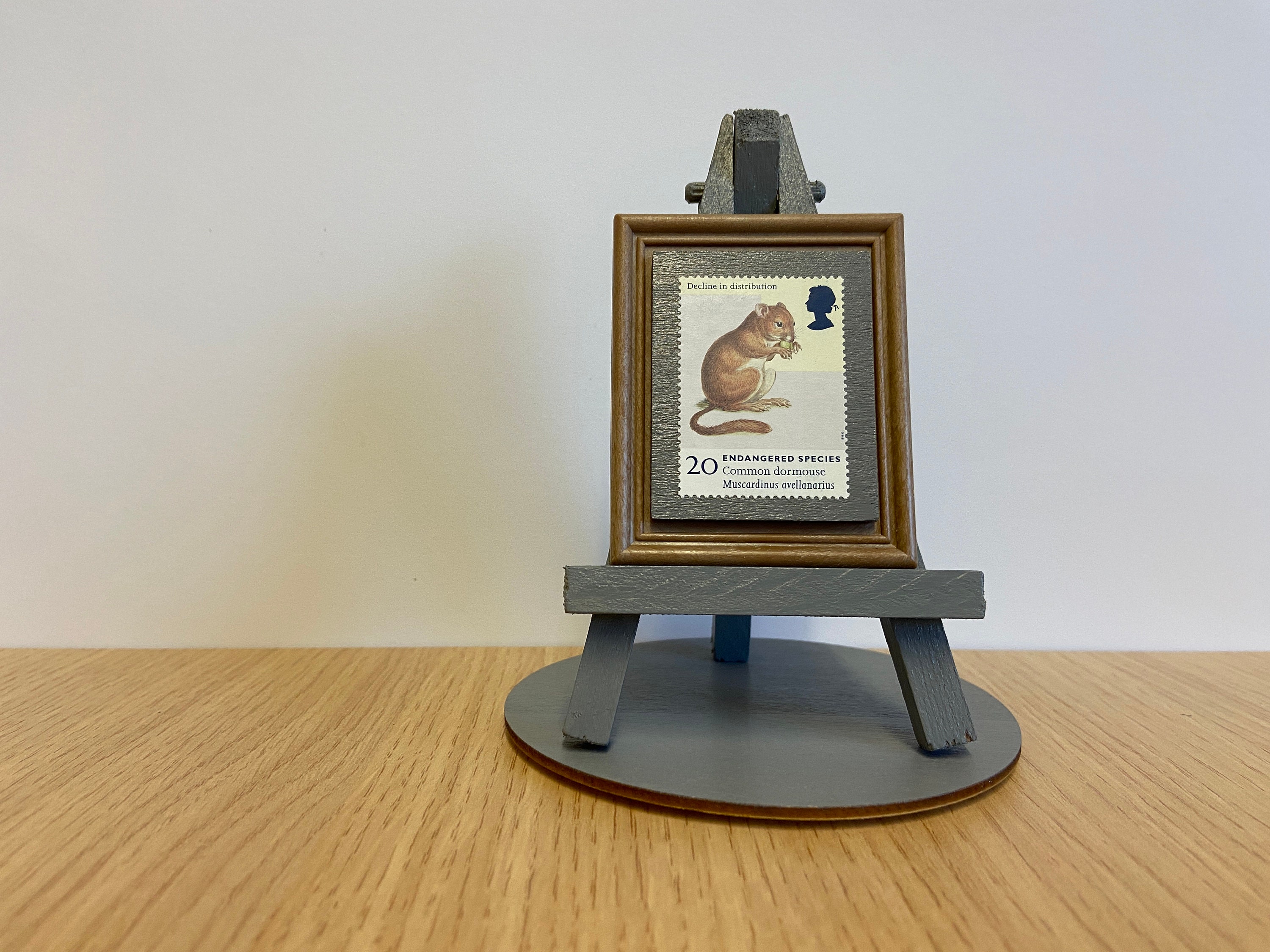This photograph depicts a miniature display setup featuring a framed postage stamp, elegantly poised on a small, easel-like stand. The background is a smooth, white wall, contrasting with the light wooden table surface on which the display is placed. The small stand, constructed of wood and painted a medium gray tone, sits upon a matching circular base, also gray with dark brown edges, giving it a classical touch.

The diminutive frame, with its dark brown wooden edges, encases the main attraction: an old letter stamp preserved with care. The stamp presents a detailed illustration of a common dwarf mouse, labeled "Endangered Species" with its scientific name "Muscadinus avelinaris." The mouse, portrayed in hues of dark and light brown, appears to be holding something close to its face, possibly nibbling on it. Its bushy tail curves gracefully towards its feet, which rest on a gray flooring within the stamp's design. 

Also featured within the stamp is the black silhouette of a woman’s head, looking left, accompanied by hard-to-read small text at the top. The bottom of the stamp clearly displays "20," signifying its denomination. The intricately frilled edges of the stamp add a vintage charm to the display, enhanced by the gentle shadows cast onto the white wall from the miniature easel.